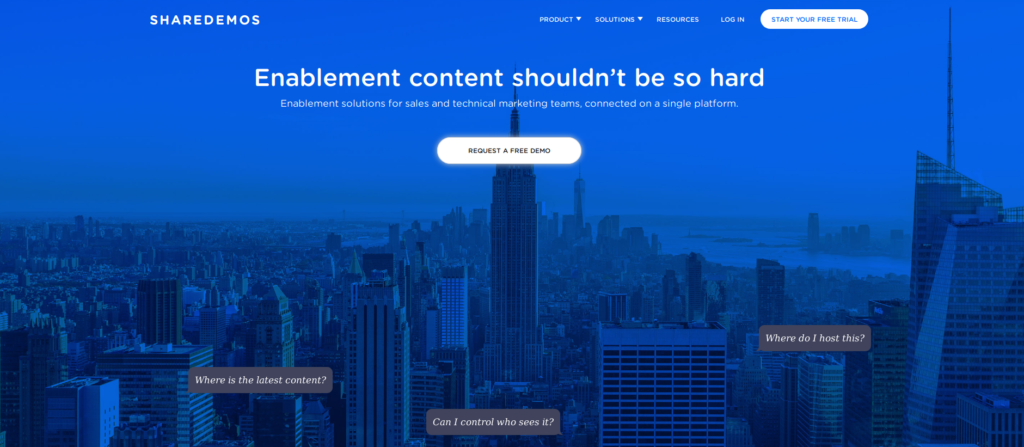A detailed description of the image presented:

The image showcases a polished and sleek website or software interface designed for a computer, developed by Shared Demos. The website's text is presented in all caps and white, unified in a single-word format. The top navigation bar has tabs for different sections: "Products," "Solutions," "Resources," "Login," and a prominent "Start Your Free Trial" button.

Dominating the center of the page is the company's motto, "ENABLEMENT CONTENT SHOULDN'T BE SO HARD," highlighted in large text. Below this, in smaller text, it elaborates: "Enablement solutions for sales and technical marketing teams connected on a single platform." A "Request a Free Demo" button is prominently placed beneath this message.

A visually appealing computer-generated image of New York City fills the background. It features a panoramic view of mid-Manhattan with the Empire State Building at the center, stretching to the southern tip of Manhattan, and encompassing the Hudson River and the ocean beyond.

At the bottom of the page, there are interactive questions addressing common concerns such as "Where's the latest content?", "Can I control who sees it?", and "Where do I host this?". Each question has a clickable button that invites users to learn more.